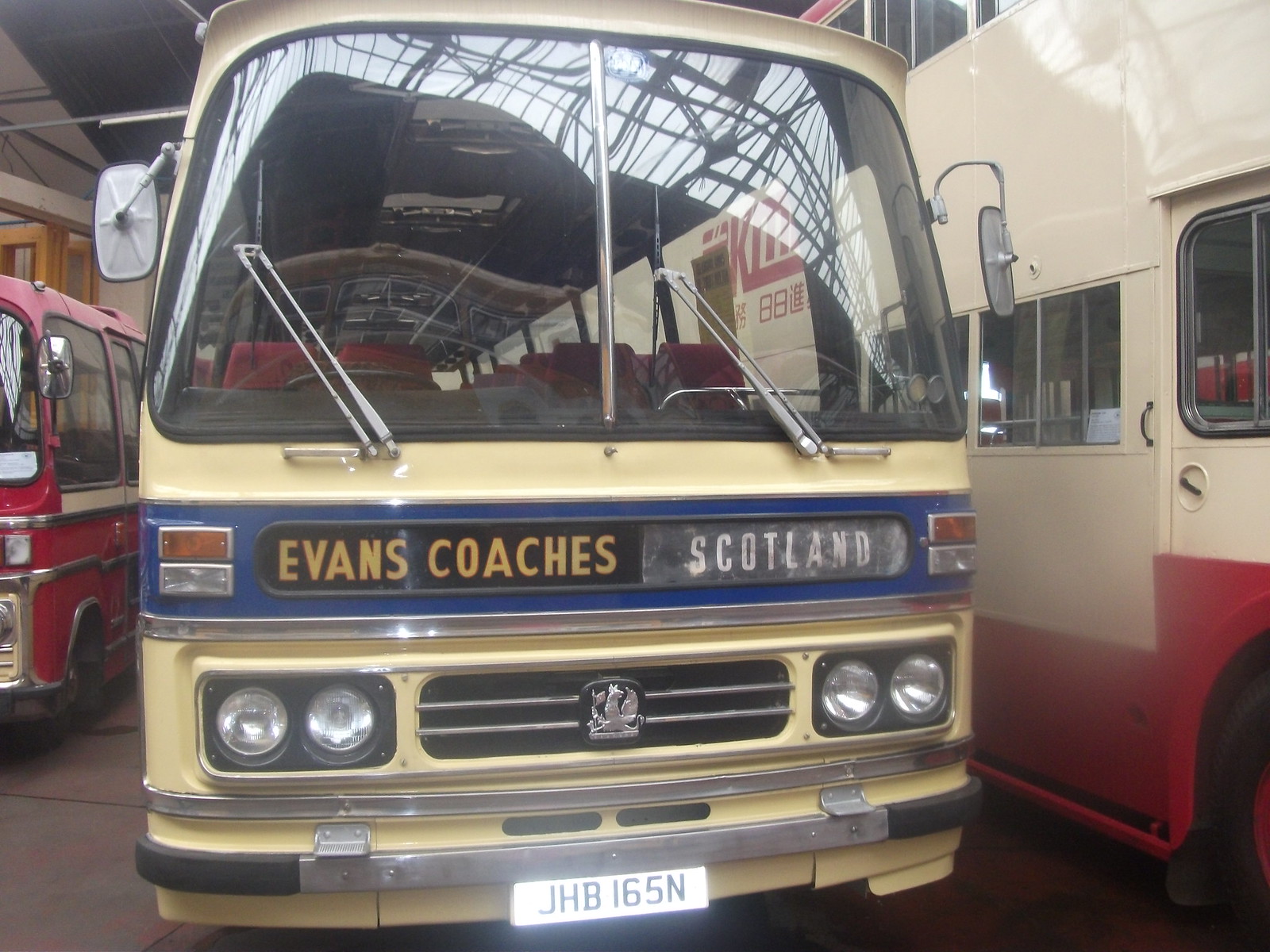The image captures a detailed scene inside a garage, focusing predominantly on the front of a yellowish-tan bus with a distinct European design. The bus, labeled "Evans Coaches Scotland" with a registration tag reading "JHB 165N," features large, curved windshield windows with two prominent, upward-angled windshield wipers and white side mirrors flanking the front. Additionally, circular headlights are visible on either side of the grille, and a blue stripe runs across the middle. On the left side of the image, a red bus with large windows is parked, while on the right, there is a food stand truck with sliding windows showcasing various cups and containers inside. The setting, illuminated by indoor lighting, appears to be a warehouse or garage, as suggested by the visible roofing structures at the top. The scene is rich in color, featuring hues of red, blue, orange, brown, white, pink, and silver in various elements throughout the composition.